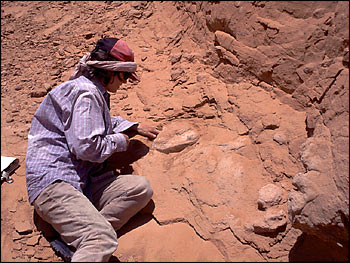This is a daytime, outdoor color photograph depicting a person, likely an archaeologist or paleontologist, engaged in excavation work amidst a rugged, red-orange rocky terrain. The individual is lying on their side, propped up on one arm on the left side of the image, with their back towards the left and their body angled towards the right. Their attention is focused downwards, carefully examining or manipulating a rock which might contain a fossil.

The person is dressed in a blue, collared button-down shirt featuring thin white vertical stripes, paired with khaki pants. They wear a head covering that includes a red and black baseball cap with a white piece of fabric tied around its back, presumably for sun protection. Scattered near the person, particularly behind them, is a large book or a stack of papers. The rocky environment is chipped and chiseled, indicative of ongoing excavation or study. The photograph captures the essence of fieldwork, framed beautifully by the bright sunlight that enhances the red hues of the sandstone surroundings.